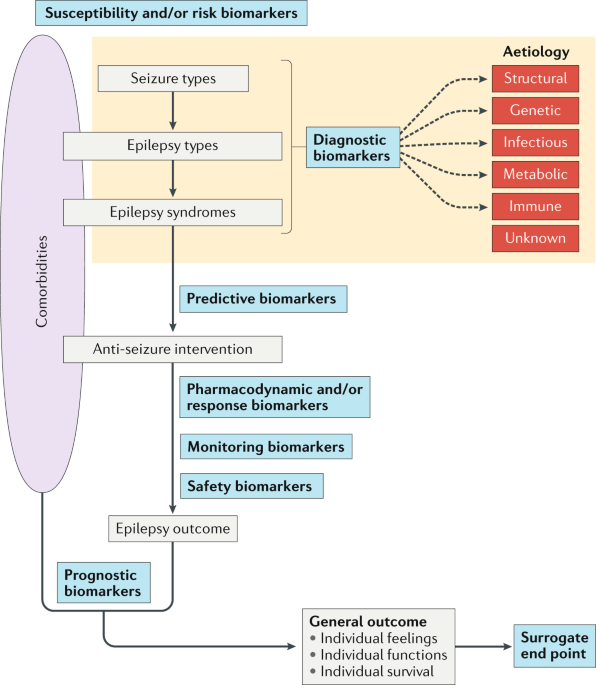The diagram intricately details the relationships between various biomarkers associated with epilepsy. Positioned at the top is the title "Susceptibility and/or Risk Biomarkers." On the left side, a purple-circled section labeled "Comorbidities" leads to a series of interconnected grey boxes with black text. These boxes sequentially represent "Seizure Types," "Epilepsy Types," "Epilepsy Syndromes," "Anti-Seizure Intervention," and "Epilepsy Outcome." Each of these elements is interconnected through arrows, illustrating a flow from one to the next.

The "Epilepsy Outcome" box has arrows leading to "Prognostic Biomarkers" with a blue background. This subsequently branches into sections detailing "General Outcome," "Individual Feelings," "Individual Functions," and "Individual Survival." All these pathways converge toward a blue box titled "Surrogate Endpoint," marking the culmination of the outcomes and interventions.

Additionally, from "Seizure Types," an arrow points toward a section on the right for "Diagnostic Biomarkers." This section, represented by red squares with white lettering, includes various categories such as "Etiology," "Structural," "Genetic," "Infectious," "Metabolic," "Immune," and "Unknown."

Overall, the diagram is a comprehensive control flow chart depicting how different biomarkers and categories interplay in the context of epilepsy, from initial seizure types to eventual outcomes and endpoints.